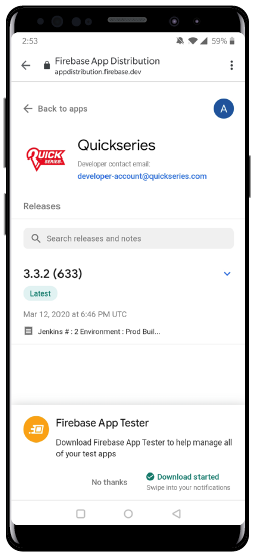**Caption:**

This image is a detailed screenshot of a mobile phone, showcasing a series of interface elements related to a Firebase application. The phone itself features a black bezel at the top and bottom, with four small circles resembling cameras, accompanied by additional sensors including a possible microphone.

At the top of the screen, the status bar displays the time "2:53" on the left, and various icons on the right: a muted alarm bell, a full Wi-Fi signal, a complete mobile signal with 59% battery remaining, and a half-full battery icon.

Below the status bar, an array of interface elements is neatly arranged:

1. A back arrow icon to the left.
2. A padlock icon beside the text "Firebase App Distribution" and its URL (partially blurry).
3. Three vertical dots aligned on the right, indicating more options.

A grey separator delineates the next section, which includes:

1. Another back arrow with the text "Back to apps" on the left.
2. A blue circle with a white capital "A" on the right.

Further down, there’s a red icon featuring a slanted question mark resembling a "Q," labeled "Quick Series." Next to it, the text "Quick Series, developer contact email" is followed by an email address "developer@quickseries.com."

A grey line separates this part from the "Releases" section, which includes:

1. A grey search bar with a magnifying glass icon, labeled "Search releases and notes."
2. Version "3.3.2" in brackets to the left of "6.3.3" and a downward arrow on the right.
3. A green "Latest" button beside the text "M8R 12, 2020 at 6:46 PM UTC."
4. A lengthy, partially obscured text starting with “Jenkins hash: 2 environment prod build” followed by an ellipsis.

Another grey line follows, leading to a more pronounced grey line with shadow effects, under which there is:

1. A label "Firebase App Tester" next to an orange circle icon on the left.
2. A prompt to "Download Firebase App Tester" for managing test apps, with options "No thanks" and a green circle with a checkmark labeled "Download started, swipe into your notifications."

At the bottom, the three navigation icons (square, circle, and left-facing triangle) conclude the image. The overall background of the screenshot is white, providing a clean and organized view of the app interface.